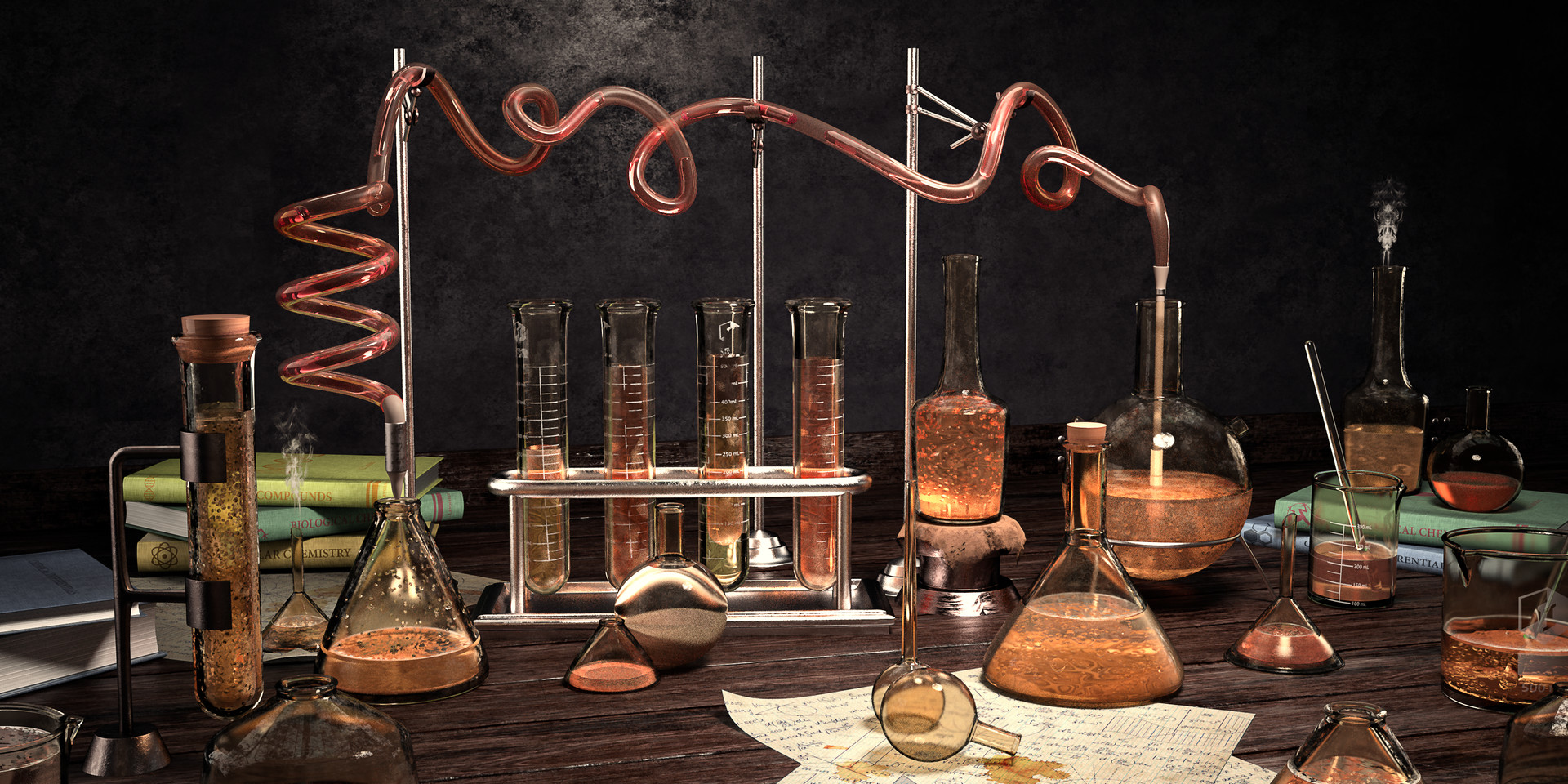The image depicts a quintessential chemistry lab scene, brimming with the quintessential tools and paraphernalia that define the discipline. Central to the image is a well-worn wooden table, dark and grainy, laden with a myriad of scientific instruments. Erlenmeyer flasks, some sealed with corks and others connected to an intricate network of hoses, sit alongside delicate glass stirring rods and an assortment of beakers. Four large test tubes are neatly organized within a test tube holder, standing upright like silent sentinels of science.

An atmosphere of activity is palpable, with wisps of steam curling upwards from the top of the image, hinting at a bubbling experiment in progress. A particularly striking detail is a flask positioned in the lower left corner, expelling steam through its narrow neck. Nearby, an assortment of books is piled haphazardly, their spines clearly marked with titles such as "Chemistry" and "Inorganic Chemistry," suggesting a rich source of reference material.

Scattered papers, filled with the scribbled notes and observations of a diligent chemist, cover parts of the table. One round-bottom flask, having tipped over, has spilled a solution onto these notes, adding a touch of chaos to the otherwise analytical setting. Clamps and mounting brackets hang off the edges of the table, ready to secure various experiments.

In the background, to the lower left, lies a booklet intended for jotting down additional notes or lab results. The backdrop of the scene is a stark black, providing a dramatic contrast that highlights every detail on the scientist's table, capturing the essence of a busy and resourceful chemistry lab.